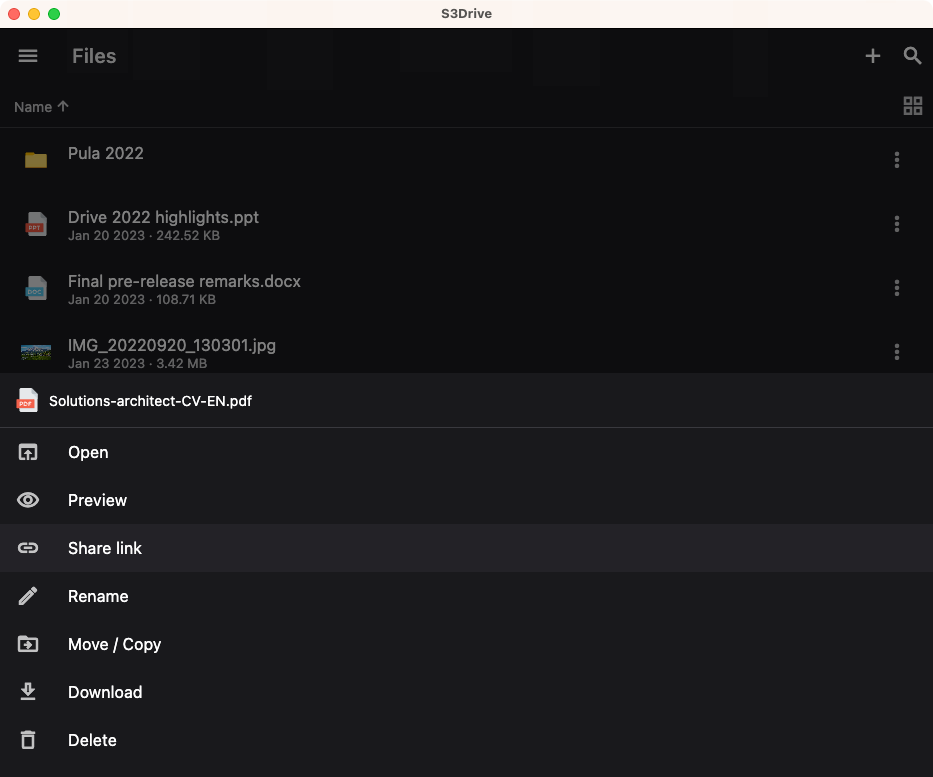The screenshot depicts a section of a website with a sleek, dark-themed user interface. The upper half of the background is black, while the lower half is a very dark gray. In the top left corner, three gray horizontal lines signify a navigational menu, with the label "Files" next to it. On the upper right side, there are two light gray icons: a search icon represented by a small circle and a plus sign.

On the left side, a column labels the category "Name," followed by a list of files, each accompanied by an icon on the left. The first item, labeled "Pula 2022," has an icon resembling a manila folder. Following this, the next file is named "Drive 2022 highlights.ppt," dated January 20th, 2023, and sized at 242.52 kilobytes. The list continues with similar details for each file.

In the section where the background transitions to light gray, a file named "solutions-architect-cv-en.pdf" appears highlighted in white font, indicating it has been selected. Below this file, a list of actions is displayed: Open, Preview, Share Link, Rename, Move/Copy, Download, and Delete, each represented by corresponding icons. For example, the Rename option features a pencil icon, the Download option shows an arrow pointing downwards, and the Delete option is symbolized by a trash can.